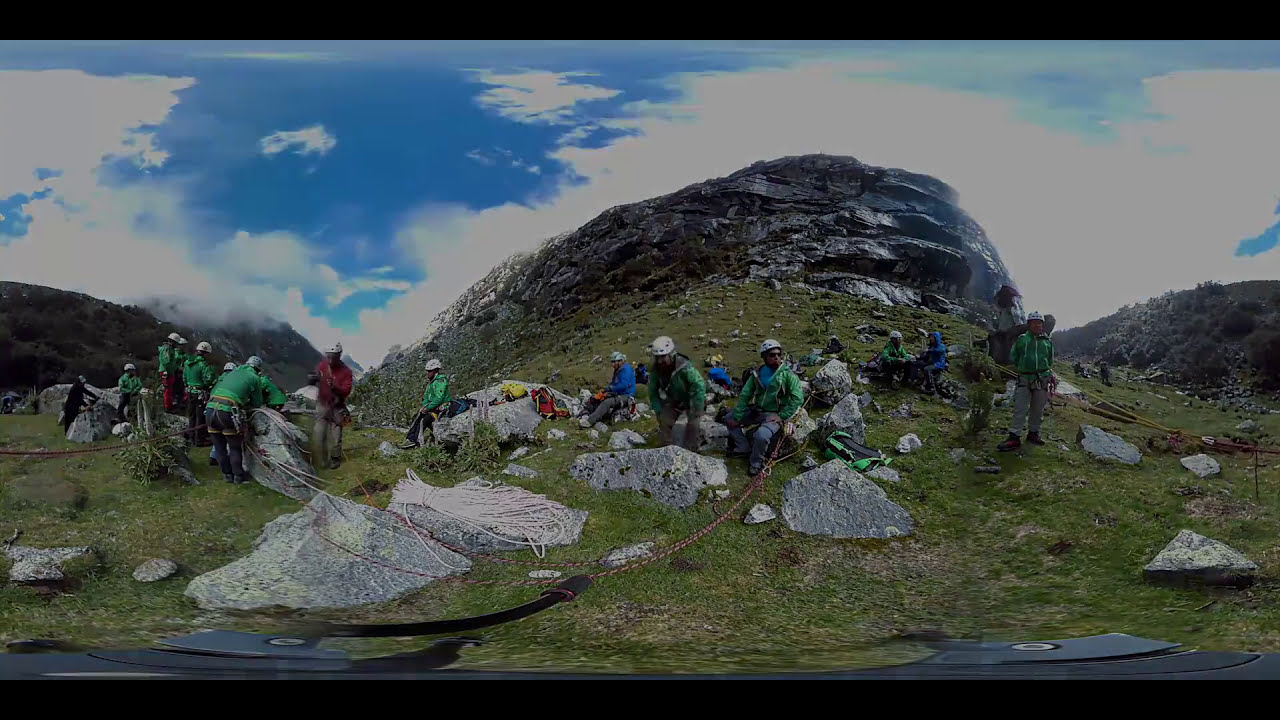This is a photograph depicting approximately 20 construction workers or mountain climbers sitting and standing on a grassy, rocky hill. Most of the individuals are wearing green windbreakers and white or silver helmets, while a few wear blue windbreakers and no helmets. They are equipped with various colored ropes, including orange, black, white, and red, which they seem to be organizing. The rocky terrain features a mix of jagged and rounded granite protrusions amidst the grass, indicative of a high-altitude, mountainous area. The backdrop includes distant, grass- and rock-covered peaks, with some extending through the clouds, highlighting the elevated location. The sky above is blue with scattered white clouds. The image has a thin black border at the top and bottom, and the colors are somewhat muted, suggesting either cloudy weather or low light conditions, all contributing to the outdoor, rugged environment the workers find themselves in.